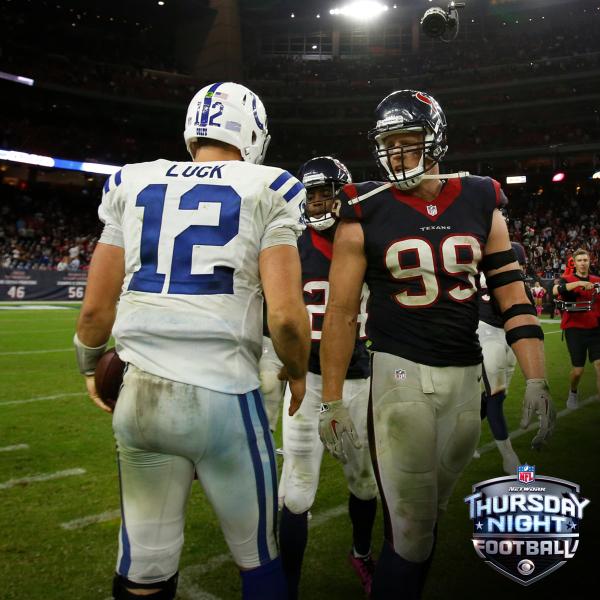The image is a vertical rectangular photograph capturing the intensity of a Thursday Night Football game. Dominating the scene are two prominent players: on the left, Andrew Luck from the Indianapolis Colts, wearing a white jersey adorned with two blue shoulder stripes, white pants with black side stripes, and a white helmet. His name, "Luck," and the number "12" are visible on the back of his uniform. To his right is a player from the Houston Texans, dressed in a black jersey with red accents on the neck and shoulders, numbered "99", and paired with white pants featuring black stripes. These players are facing each other amidst a bustling stadium filled with spectators, illuminated by bright lights overhead. Additional figures populate the background, including a game official and a cameraman in red. In the lower right corner, the NFL Network Thursday Night Football logo is prominently displayed, bordered by a shield with "Thursday Night" in blue and "Football" in silver, accompanied by the NFL emblem at the top.